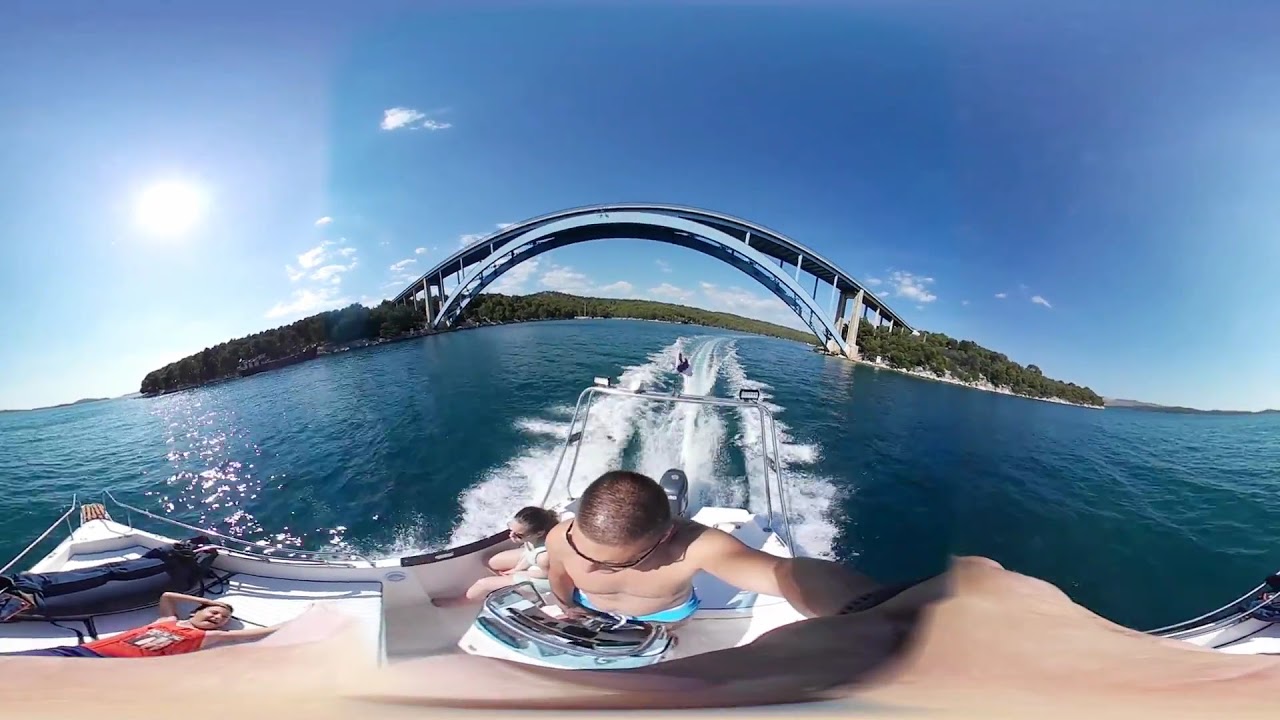The image captures a dynamic scene on a speedboat navigating a large, tranquil body of water under a bright, mostly clear blue sky. At the forefront of the image, a man, shirtless with short brown hair and wearing sunglasses, is steering the boat with his right hand while holding a camera aloft with his left, suggesting a sense of adventure and spontaneity. The man is dressed in blue shorts and stands against the boat's controls, focused on navigating through the water. Beside him, a woman dressed in a white swimsuit and also wearing sunglasses, sits with her hair pulled back, gazing forward.

In front of the boat, a child wearing an orange tank top and blue shorts is laid out across the deck, seemingly relaxed with his hands behind his head. Nearby, the boat cuts through the water at high speed, evidenced by the white waves trailing behind them. They appear to be towing someone on a small raft or possibly skiing, adding to the exhilarating atmosphere of the scene.

The background features lush greenery and trees along the shoreline, with a few houses nestled among them, creating a picturesque contrast to the expansive blue-green water. Dominating the horizon is a large, arching blue metal bridge, elegantly connecting two sections of land, likely an island with mountainous terrain. The image, probably taken with a 360-degree camera, captures the vast expanse of water, the boat's passengers, and the scenic environment, encapsulating a perfect day out on the lake.